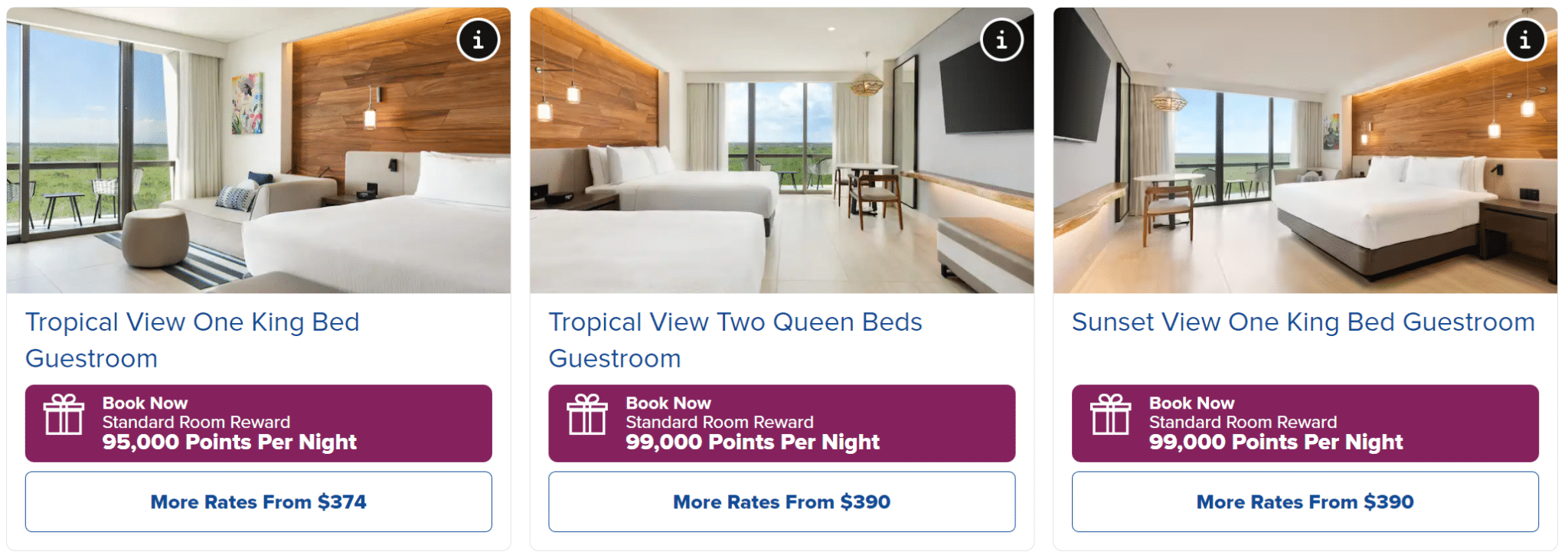The image features three individual sections, separated by white space, presenting different guest room options available at a hotel.

1. **First Section:**
   - **Image Description:** A hotel room with a wooden headboard and a neatly made white bed.
   - **Text Details:** 
     - Main Text: "Tropical View, One King Bed, Guest Room"
     - Call-to-Action Button: A purple rectangle with white text reading "Book Now, Standard Room, Reward: 95,000 points per night."
     - Additional Option: A blue-outlined white box with blue text indicating additional rates, "$374 per night."

2. **Second Section:**
   - **Image Description:** Another angle of a similar hotel room, showcasing two queen beds.
   - **Text Details:**
     - Main Text: "Tropical View, Two Queen Beds, Guest Room"
     - Call-to-Action Button: Identical purple rectangle with white text reading "Book Now, Standard Room, Reward: 90,000 points per night."
     - Additional Option: Blue-outlined white box with blue text suggesting more rates at "$390 per night."

3. **Third Section:**
   - **Image Description:** A room offering a sunset view featuring one king bed.
   - **Text Details:**
     - Main Text: "Sunset View, One King Bed, Guest Room"
     - Call-to-Action Button: Matching purple rectangle with white text reading "Book Now, Standard Room, Reward: 90,000 points per night."
     - Additional Option: Blue-outlined white box with blue text displaying more rates, "$390 per night."

Each section is clearly defined and provides a comprehensive view of the room types, rates, and points needed for booking, allowing potential guests to make an informed decision.